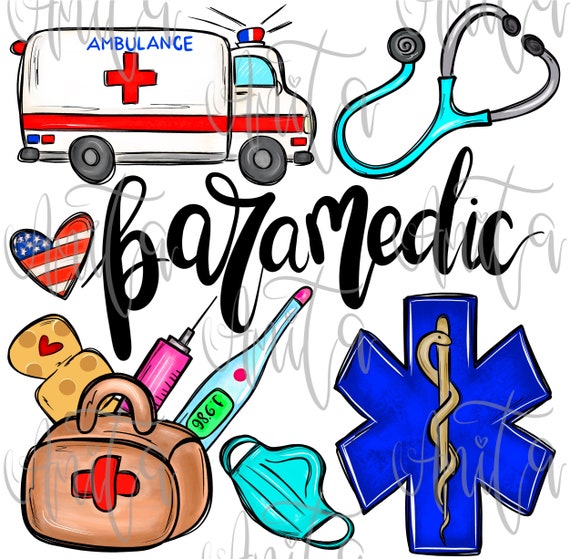The image features a detailed collection of cartoon drawings dedicated to the field of paramedics. At the center, large black cursive text reads "paramedic," emphasizing the primary theme. Surrounding this central text are various elements associated with emergency medical services: 

- An ambulance, positioned in the upper left corner, complete with a Red Cross emblem, red and blue flashing lights, a siren, and a red stripe down the middle.
- A stethoscope, found in the upper right corner, featuring a bright neon aqua-blue cord and the classic chest piece.
- A heart-shaped depiction of the American flag is set slightly off-center to the left.
- A brown medical satchel with a Red Cross is located in the lower left corner, containing a pink syringe, a thermometer, a bandage with a red heart, and other medical supplies.
- Adjacent to the satchel is a blue face mask, commonly used to prevent disease transmission.
- In the lower right corner, the medical profession's iconic symbol, the Rod of Asclepius (a gray snake entwined around a staff), is displayed.

The entire collage is surrounded by faint gray text, potentially crediting the creators. This rich assortment of images collectively pays homage to the dedication and essential role of paramedics in providing mobile treatment for illnesses and injuries.